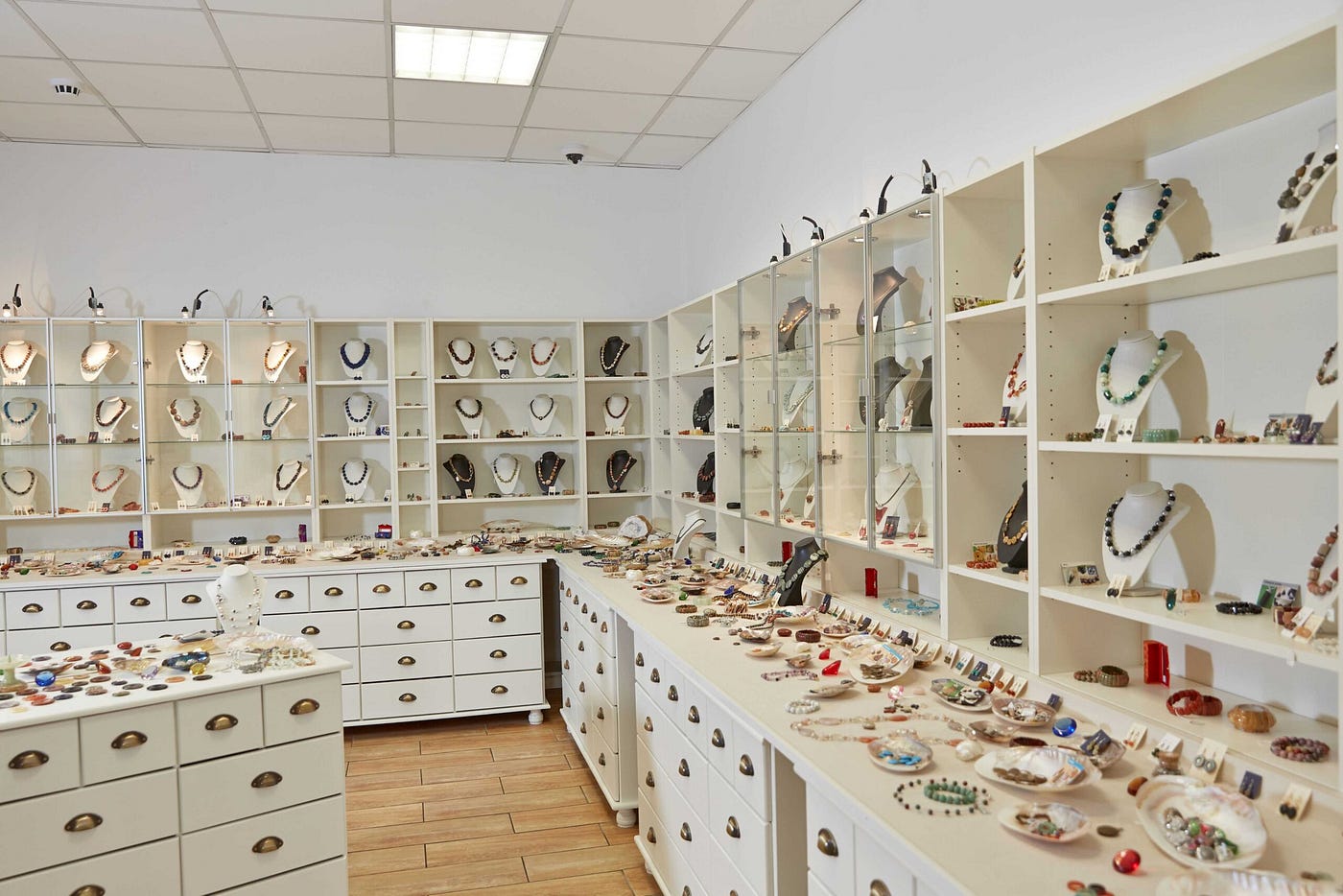The image showcases a well-organized jewelry store, primarily featuring costume jewelry. The store is designed with a clean, white-and-cream color scheme, complemented by a warm brown wooden floor and a white drop ceiling, possibly equipped with security cameras and lights. A centerpiece of white cabinetry occupies the center of the room, displaying various colorful jewelry pieces on its countertops. Along the back and side walls are several white shelves and cabinets with brass handles, some of which have doors, likely housing more valuable items. The shelves are lined with mannequin necklace holders showcasing beaded necklaces of various vibrant colors, alongside bracelets made of stones and beads. Small plates, some shell-shaped, are scattered across the countertops, further displaying an array of brightly-colored, eye-catching costume jewelry, thus underscoring the decorative nature of the items rather than their preciousness.